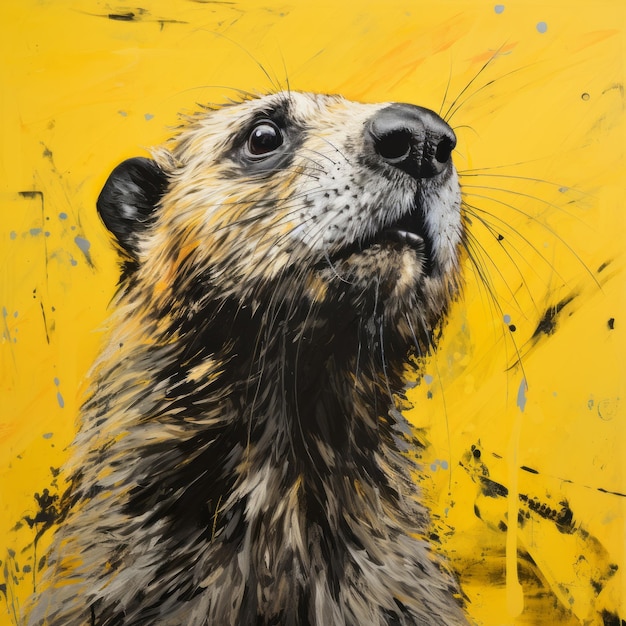This AI-generated image is a close-up portrait of a marmot-like rodent, showcasing a vibrant, hyper-realistic depiction. The animal, possibly mistaken for a beaver or woodchuck, is facing right, prominently featuring its large, shiny black nose and abundant black whiskers. Its big, seemingly startled eyes reflect light as if reacting to a sudden noise. The fur around its muzzle is white, while the rest of the coat varies in dark and light brown, with shades of gray. The little brown or black ears add to its endearing appearance. The creature is set against a bright, taxi cab yellow background, resembling the bustling hues of New York City. The backdrop is further embellished with dramatic splashes and splotches of black, gray, and dripping yellow, adding an abstract and dynamic feel to the composition.